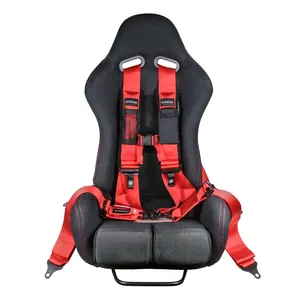The image is a detailed product photograph of a black ergonomic racing seat designed for automobiles, likely showcased on a retail website. The seat features a tall, contoured backrest with a sleek, black, futuristic design, including two gray cushions at the bottom section. Prominent red harness straps, reminiscent of heavy-duty racing seat belts, emerge from two holes near the top center of the seat. These straps cascade over the shoulder area and then connect to additional red straps that secure across the waist. The lap belt is shown draped over the armrests, lying spread apart to either side in an open position, emphasizing the intricate harness system. Additionally, the seat has two armrests and a distinctive bucket-style construction, all set against a plain white backdrop for a professional product presentation.